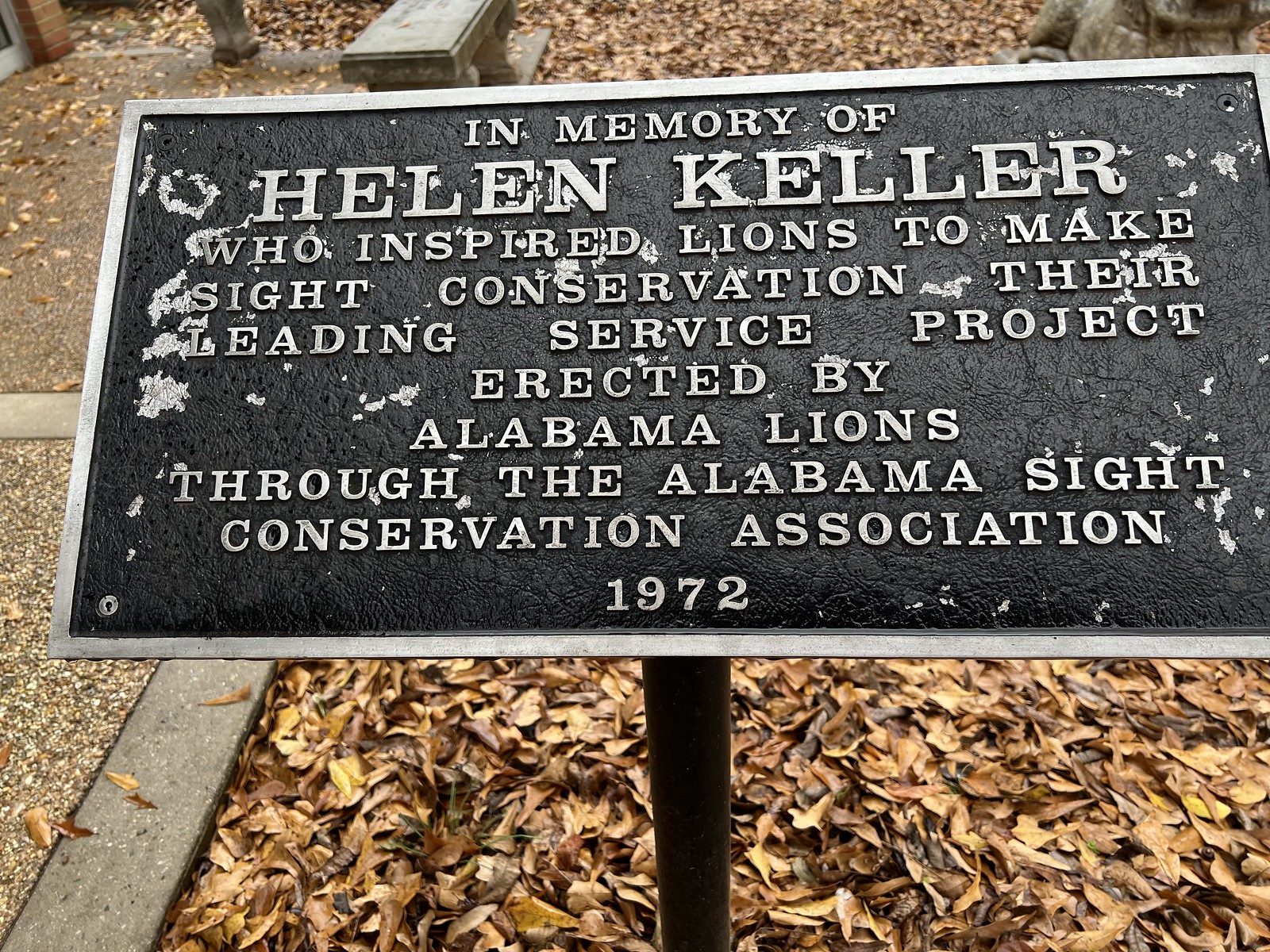The image depicts a memorial plaque dedicated to Helen Keller, mounted on a pole approximately three to four feet above the ground. This black plaque features a gray border and etched text that reads: "In memory of Helen Keller, who inspired Lions to make Sight Conservation their leading service project, erected by Alabama Lions through the Alabama Sight Conservation Association, 1972." The plaque appears weathered, with some parts showing minor chips and fading. Situated in an outdoor park-like reflection area, the setting is characterized by a ground layer of fallen leaves, indicating a fall season. To the left of the plaque, there is a mixture of concrete and gravel paths, while toward the back, a reflection bench is visible, offering a serene spot for contemplation.